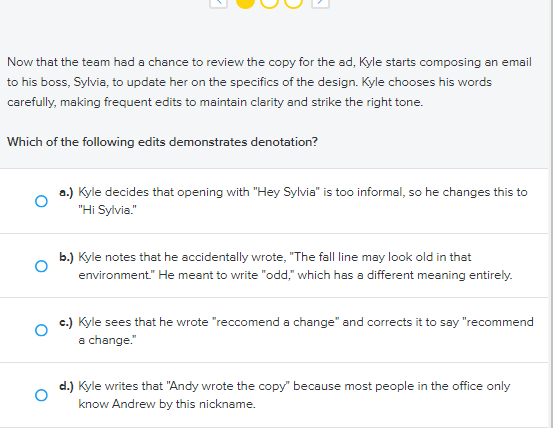The image depicts a multiple-choice question. At the top, there are three yellow bubbles, with the first bubble highlighted to indicate the current question. The question itself is displayed in dark gray or black text within a gray bar at the top of the section, which stands out against the lighter gray background. 

The text reads: "Now that the team has had a chance to review the copy for the ad, Kyle starts composing an email to his boss, Sylvia, updating her on the specifics of the design. Kyle chooses his words carefully, making frequent edits to maintain clarity and strike the right tone. Which of the following edits demonstrates denotation?"

Four options are listed below the question, each without any selection marked:
A. "Kyle decides that opening with 'Hey, Sylvia,' is too informal, so he changes it to 'Hi, Sylvia.'"
B. "Kyle notes that he actually wrote 'the form,' but he meant to write 'odd,' which has a different meaning entirely."
C. "Kyle sees that he wrote 'recommend a charge,' and he corrects it to 'recommend a change.'"
D. "Kyle writes that 'Andy wrote the copy' because most people in the office only know Andrew by his nickname."

The purpose of the question is to identify which of these edits best demonstrates the use of denotation, which refers to the explicit or direct meaning of a word.